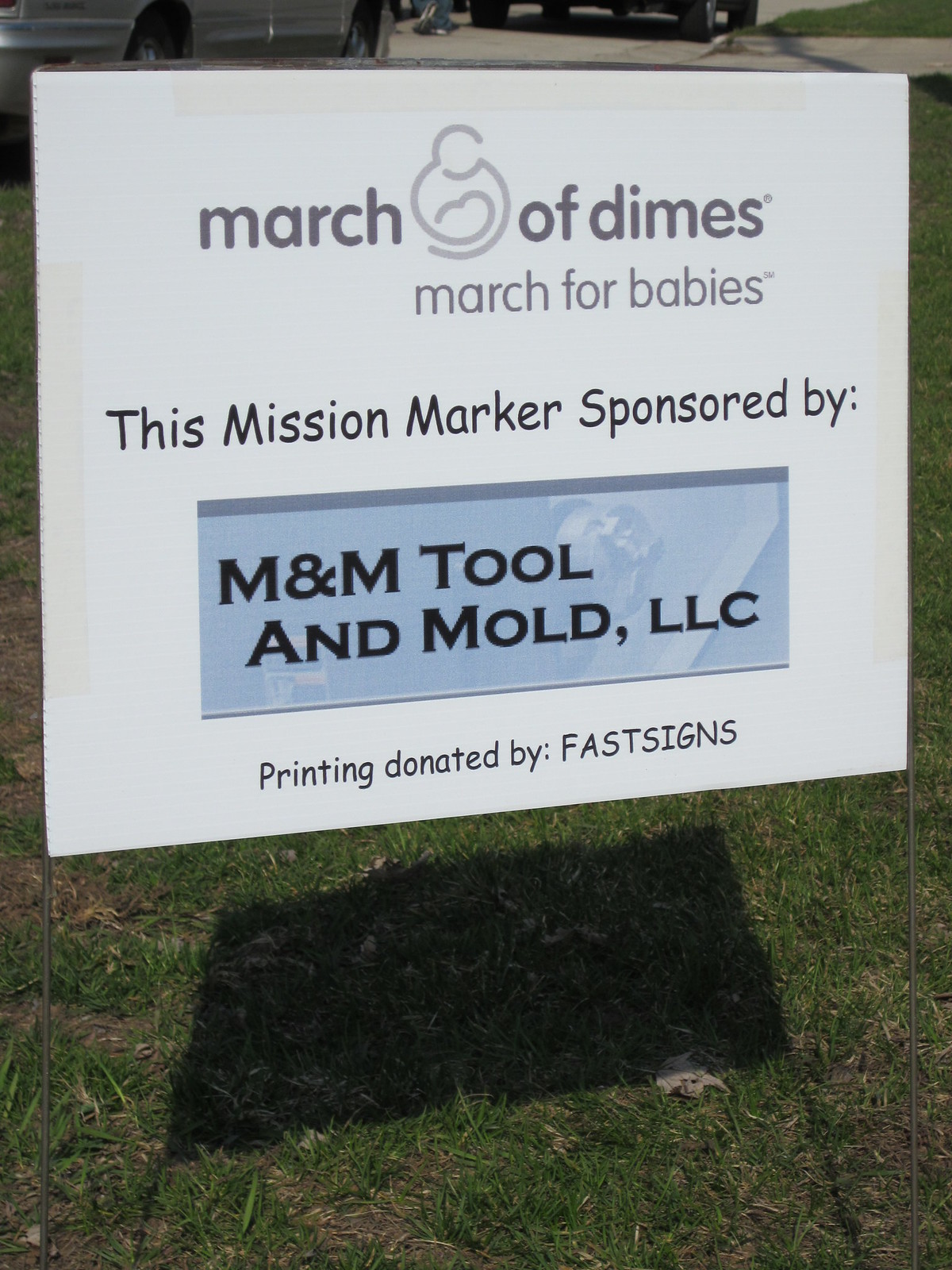This outdoor sign, staked into the grass on two metal poles, is a white printed marker for the March of Dimes charity. The sign reads, from top to bottom: "March of Dimes," with the emblem of a woman and a baby placed between "March" and "Of." Below it in slightly lighter print is "March for Babies." Further down, the sign states "This Mission Marker, Sponsored By," followed by a silver and blue rectangle containing the text "M&M Tool and Mold, LLC" in black. At the bottom, it says, "Printing Donated By Fast Signs" in all capital letters. The grass beneath the sign is patchy, with both green areas and brown dirt visible. The sun casts a shadow of the sign onto the ground behind it, indicating it's a bright, sunny day. In the background, there are some indeterminate objects.